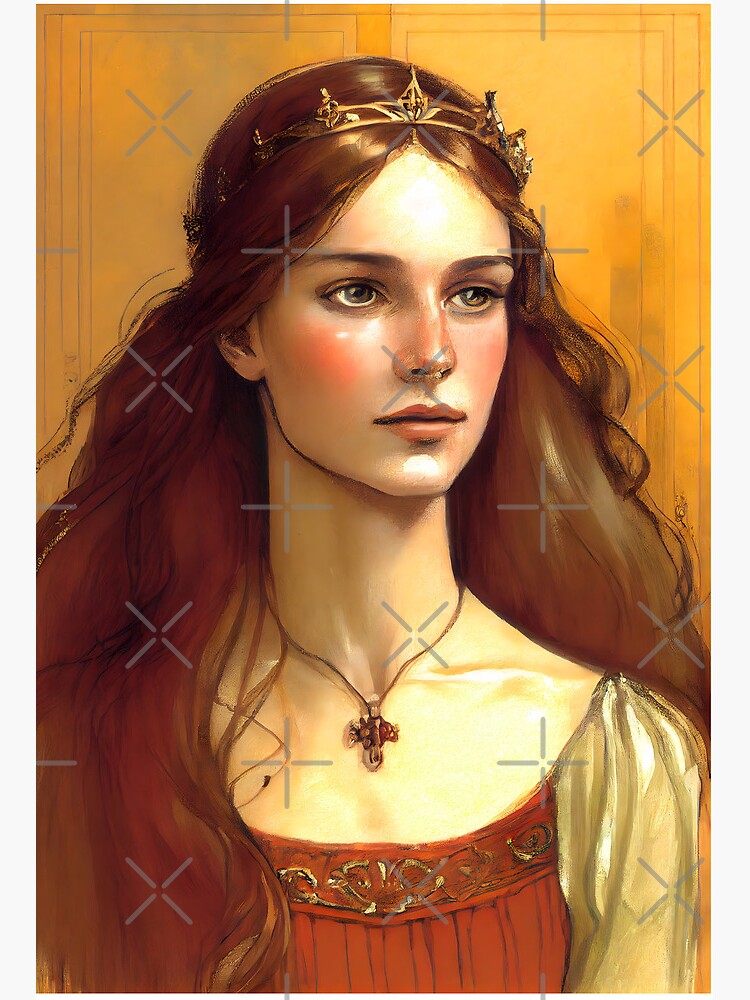The image depicts a painting or a paint-style digital art piece of a young Caucasian woman from a medieval or Renaissance era. She has long flowing auburn hair adorned with a simple, gold diadem, and she gazes to the right of the image, showcasing her greenish-brown eyes and rosy cheeks. The woman is wearing an elaborate orange dress with puffy, possibly beige sleeves and intricate gold embroidery at the neckline, which is of a bare shoulders style. A cord or simple chain around her neck holds a vaguely cross-shaped amulet. She has a slender build and a notably long neck. The background is a golden yellow, over which a gray watermark featuring a mix of plus signs and Xs is overlaid, forming a grid-like pattern. Overall, while the artwork is not highly advanced, it effectively captures the elegance and poise of its subject.